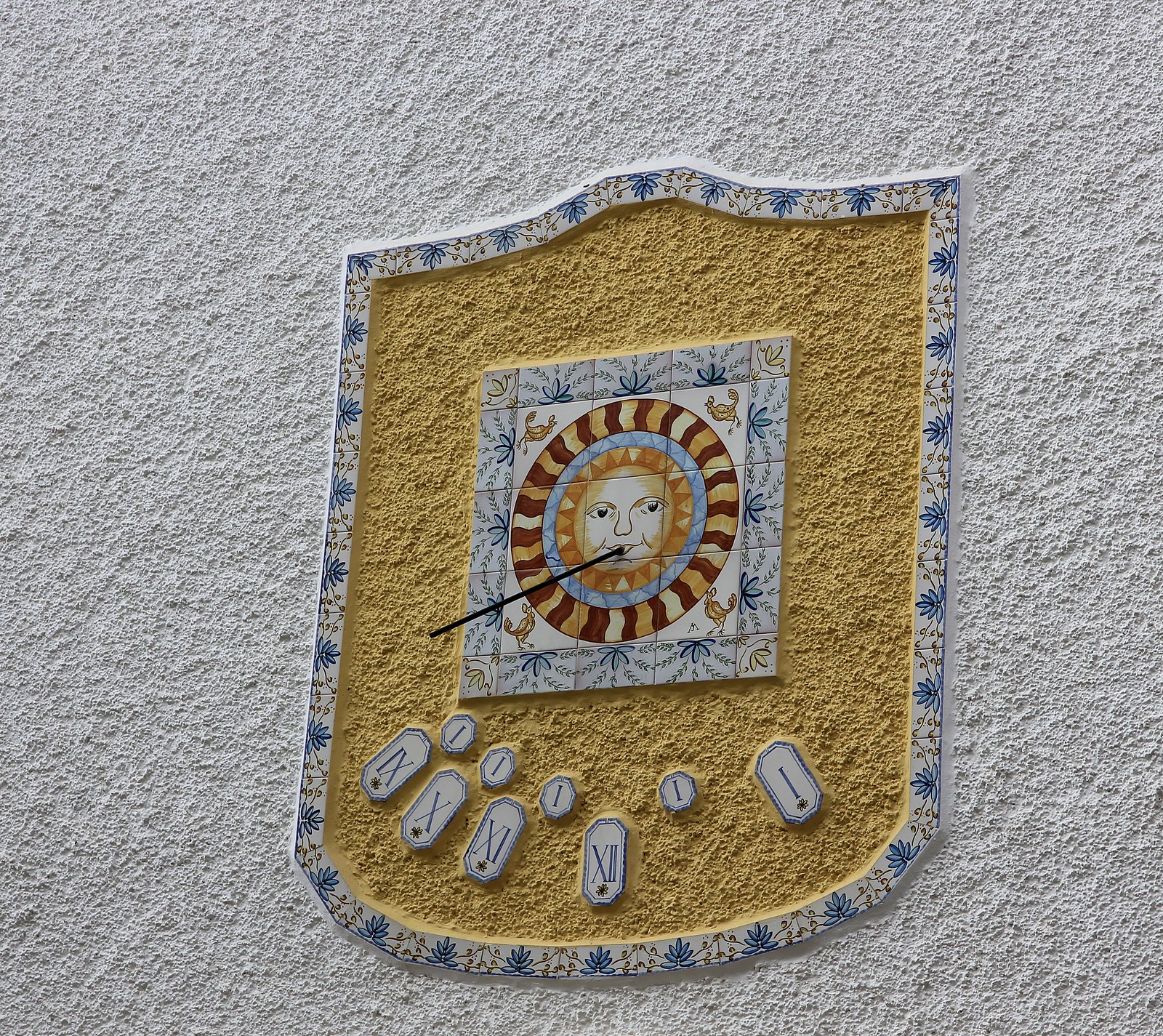This image showcases a decorative stone wall with a textured, white popcorn finish. Prominently featured in the center of the wall is a detailed, crest-shaped ornament that evokes the form of a shield. The crest has a distinctive shape, being rounded at the bottom, squared on the sides, and slightly indented at the top. It is bordered by a mosaic of white tiles adorned with blue flowers and brown vines, adding an ornamental touch to the design. Within this border is a mustard yellow and gold interior, which encases another square of intricately arranged tiles.

At the heart of this tiled square lies an artistic depiction of the Sun, complete with facial features that include eyes, a nose, and a mouth, out of which protrudes a black straw-like element. Surrounding the Sun's face are alternating rings of gold, blue, and multi-colored stripes, giving it a radiant appearance. The background surrounding this central motif transitions to a white area decorated with images of red roosters positioned at the four corners, adding an additional layer of detail. Below this elaborate sun motif, Roman numerals are displayed, suggesting a possible function as a sundial or a sculptural sign. The entire composition is visually rich and multifaceted, making it an engaging and intricate piece of art on the wall.